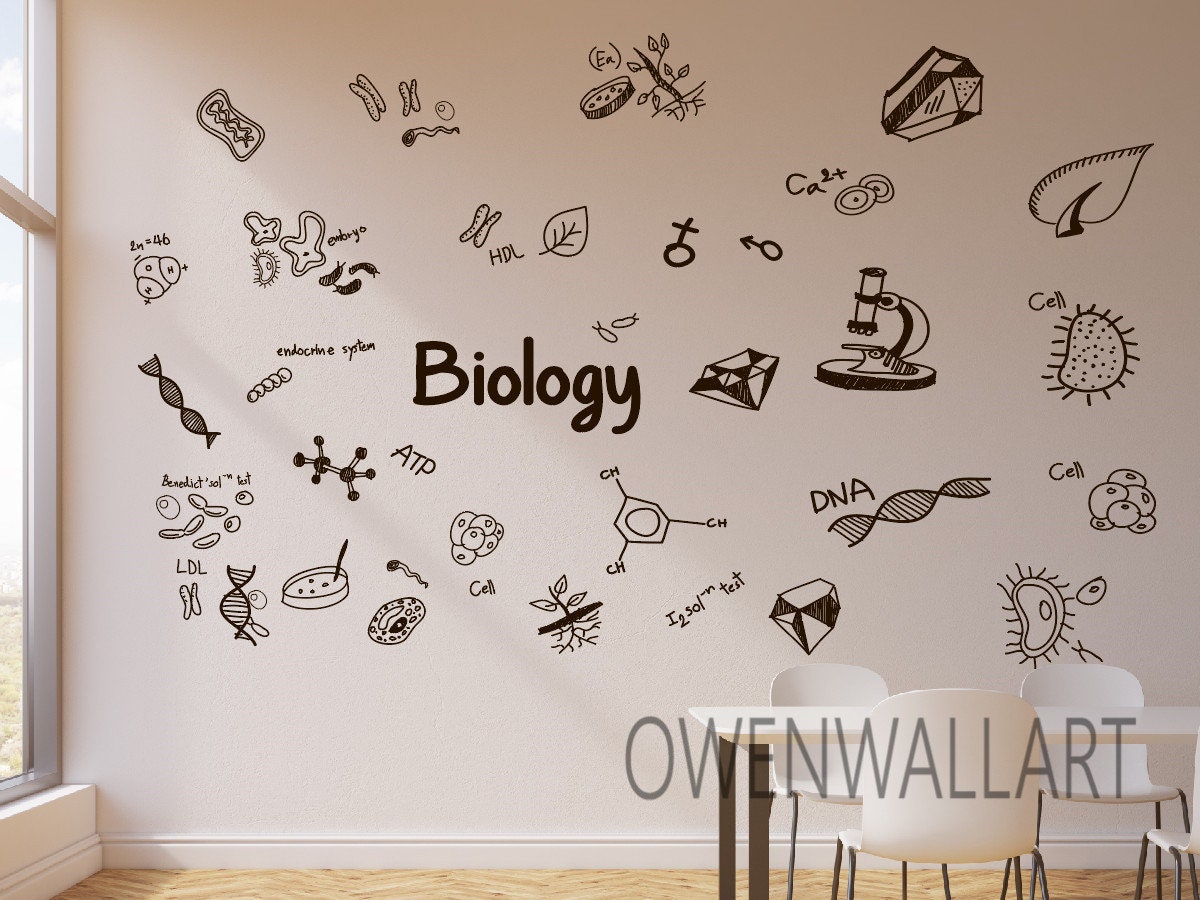The image depicts an indoor wall within a room, likely a biology classroom or study area. The wall, which is slightly beige in color, is adorned with a detailed array of black and white hand-drawn sketches and text related to biology. Prominently, the word "Biology" is boldly written at the center. Surrounding it are meticulous drawings of scientific elements such as a microscope, a DNA double helix, clusters of cells, various single-celled organisms, plant sketches, and symbols for male and female. Additionally, there are labeled text including formulas like ATP and chemical notations such as CA2+. These elements are illustrated in a manner suggesting they might be seen under a microscope, making the wall an educational canvas.

In the bottom right corner of the wall, in pale gray text, is the watermark "Owen Wall Art," confirming the artistic contribution. The image also includes a glimpse of a white table with black legs and molded plastic white chairs situated in the bottom right, indicating a possible study space. The left side of the image shows part of a window extending nearly from floor to ceiling, allowing light to potentially illuminate the detailed drawings. The entire setting exudes an educational ambiance ideal for a science classroom or lab.